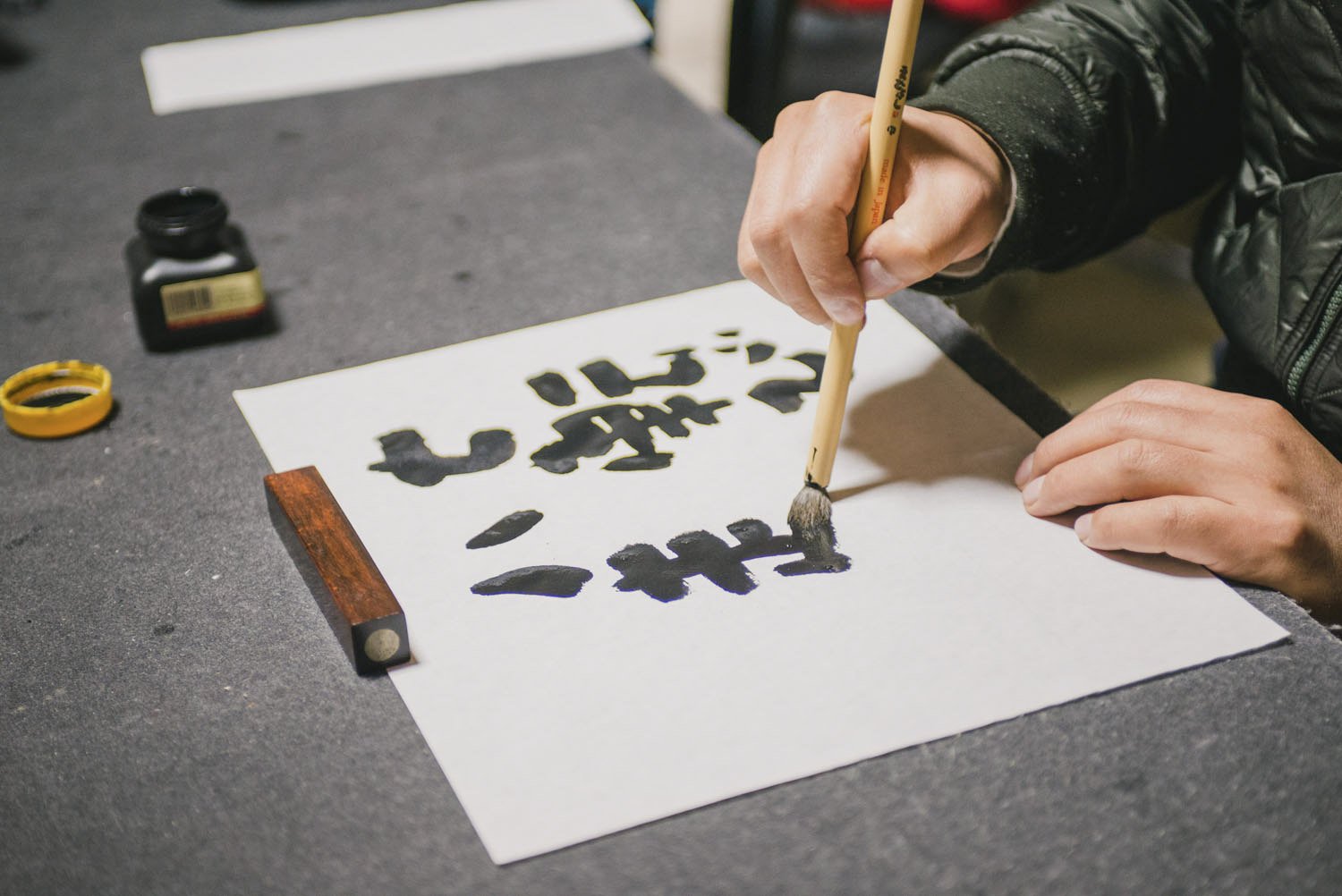In this detailed image, a right-handed individual is meticulously writing Chinese characters on a stark white calligraphy paper, positioned on a gray desktop. The paper is held in place at the top by a square piece of wood with a metal cylinder embedded in it. The person is using a large, beige-colored calligraphy brush, poised expertly over the paper. On the left upper part of the image, a black bottle of ink with a yellow label and an unscrewed yellow lid lies open, with the lid placed upside down on the table. The ink itself is black, and some additional sheets of paper can be seen in the distance. The writer, wearing what appears to be a black leather jacket, focuses on the precise formation of multiple Chinese symbols, progressing from right to left across the sheet. A slightly blurred red object can be seen behind the person's sleeve, adding to the intricate setting of the scene.